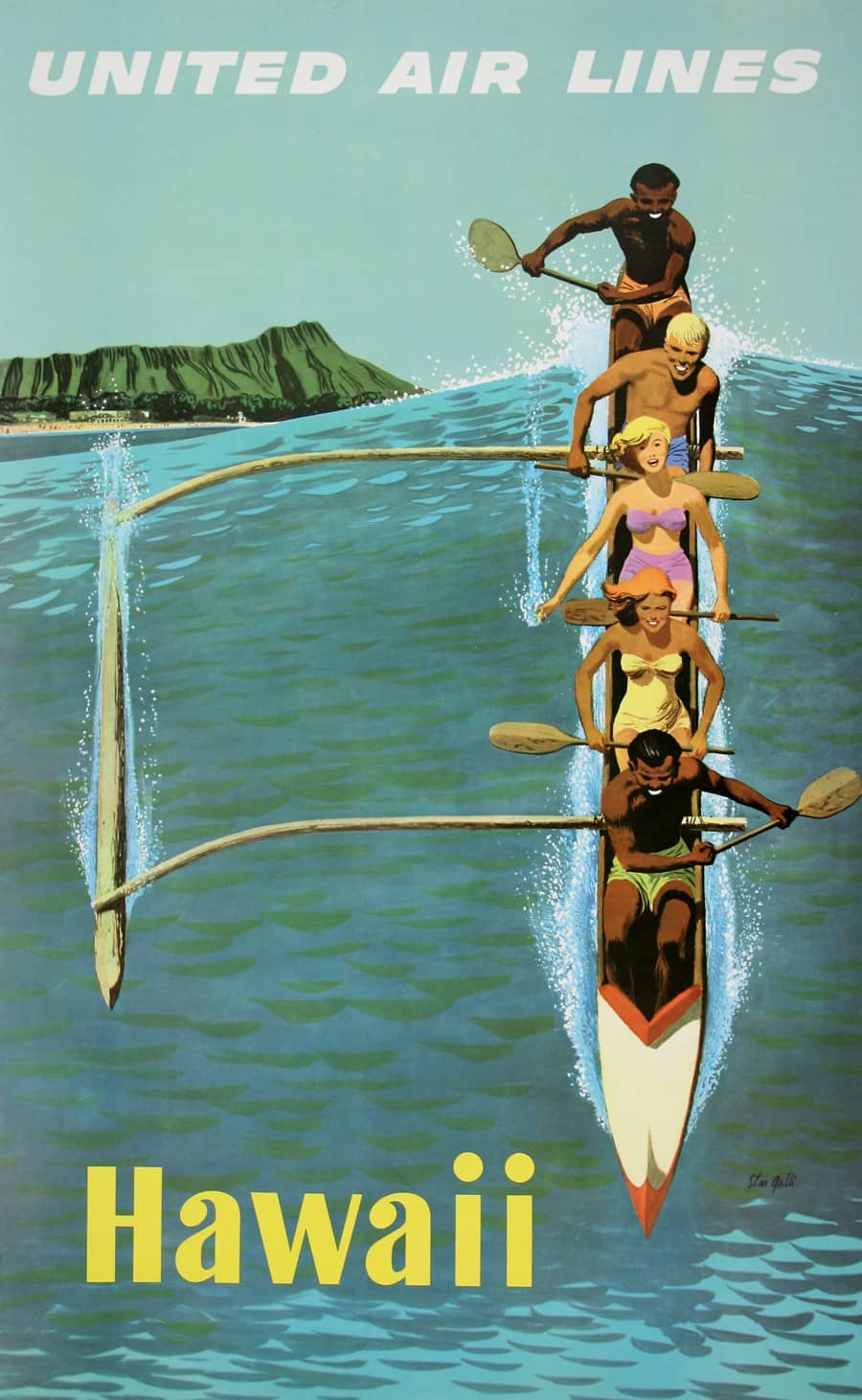This vertical vintage-style poster for United Airlines features a dynamic scene promoting travel to Hawaii. Dominated by shades of blue and green, the top of the poster displays "UNITED AIRLINES" in bold, all-caps white text set against a clear blue sky. Below, a lush green mountain ridge extends over a distant beach, framing the idyllic background. 

In the foreground, a massive, light blue and green wave curls majestically, capturing the thrilling motion of an outrigger canoe riding its crest. The white canoe, accented with orange tips, is equipped with an outrigger on its left side stabilized by wooden bars. It carries six young, smiling individuals: two Black men at either end, an overall balance maintained by a man in blue swimwear and two women at its center. One woman wears a purple bikini, the other a yellow strapless one-piece, both gripping their paddles with enthusiasm as they navigate the wave.

At the bottom left corner of the image, "HAWAII" is displayed in vibrant yellow text, underscoring the travel destination. This promotional imagery captures the adventurous spirit and scenic beauty of Hawaii, highlighting the excitement of a United Airlines journey to this tropical paradise.